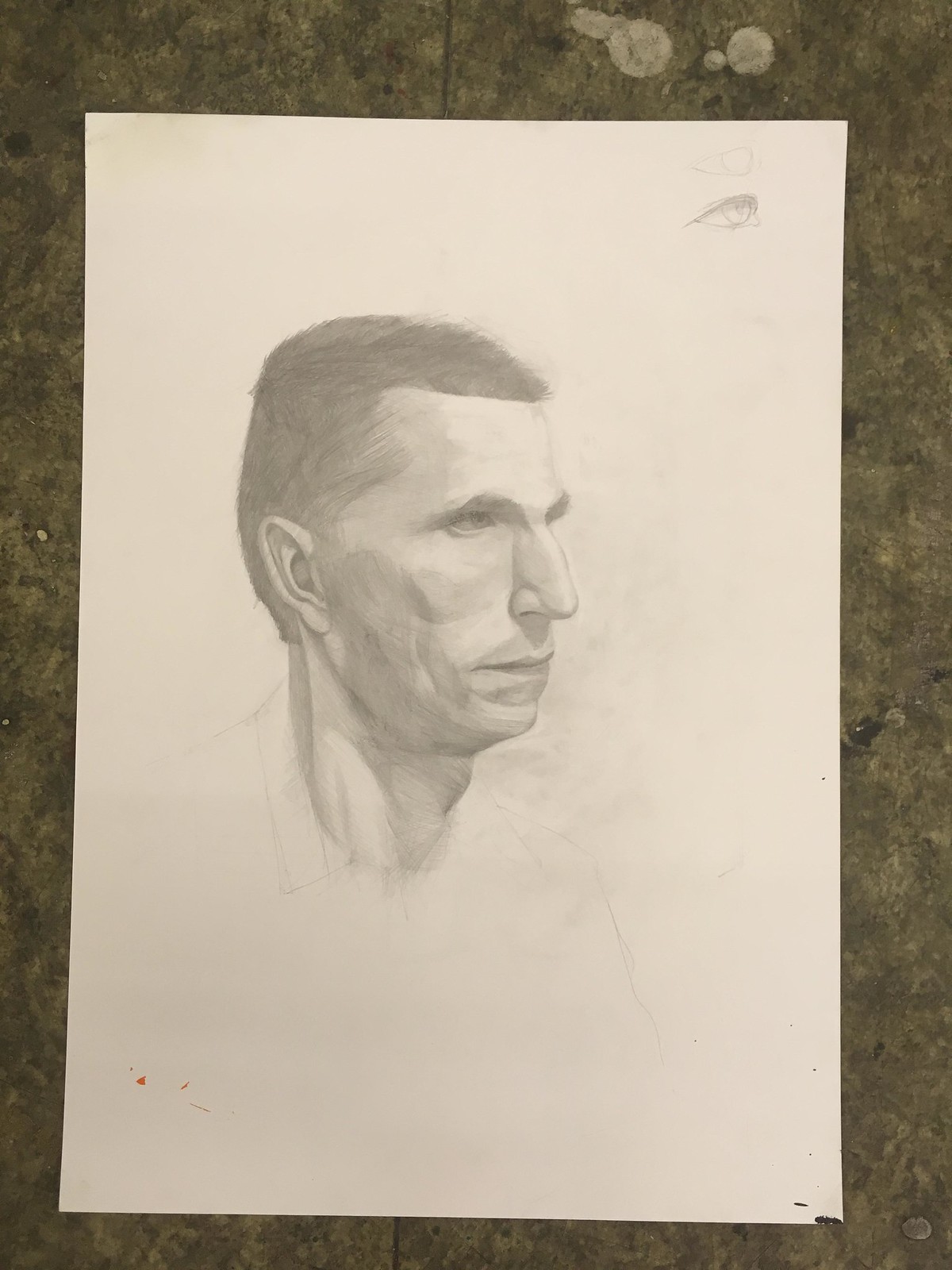A meticulously detailed pencil drawing showcases a man with a blocky, angular face, resting on a pristine piece of white paper. The paper contrasts starkly with the dark, gray, and black marble-patterned countertop it is placed upon, enhancing the drama of the scene through the somber background. The focal point of the sketch is the man's face and neck, both rendered with significant detail. His elongated, narrow oval-shaped head features small, pointed ears and a disproportionately small forehead compared to his prominent nose and mouth, creating a unique, somewhat stretched appearance. He sports a close-cropped, flat-top haircut that ends sharply at his forehead, adding to the angular aesthetic.

The man's neck is lean and angular, almost exaggerated in its form. His expression is contemplative, with one eye intriguingly inset, as if lost in deep thought. Despite his thin lips, his large mouth area and weak chin define his facial structure, while a few wrinkles and age lines suggest a slightly older age. The barest lines of what appears to be a collared shirt are faintly traced beneath his detailed head and neck, leaving the focus on the intricacies of his visage. This detailed depiction captures a visage both lifelike and abstract, blending precise realism with artistic exaggeration.